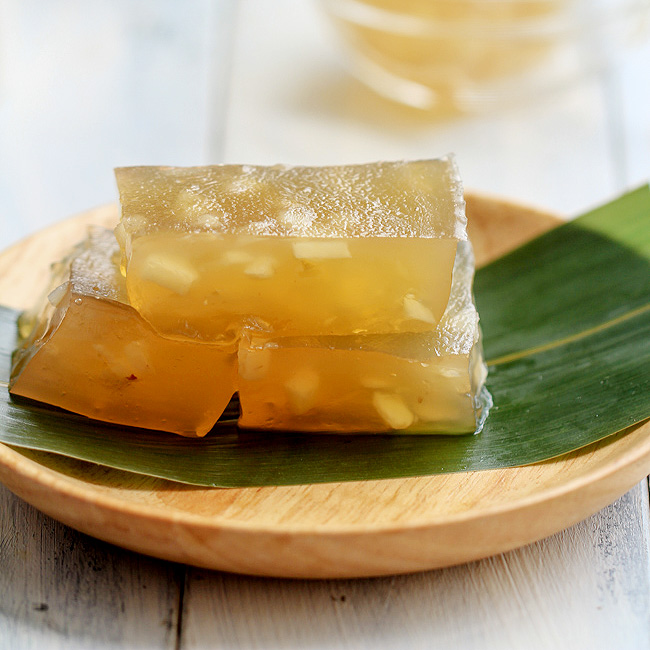The professional, stylized photograph depicts an elegant presentation of an Asian dessert. Positioned on a circular, handmade wooden plate, painted light beige-brown, a vibrant green banana leaf serves as a natural lining. Resting atop the leaf are three rectangular, gelatinous cubes of a yellowish-gold hue, slightly transparent with visible reflections of light, revealing small white bits inside, which could be pieces of fruit, nuts, or coconut, contributing to their soft texture. The plate is set on a white-painted wooden picnic table, adding a rustic charm. In the blurry background, a cup of yellowish drink or tea, its details indistinguishable, complements the aesthetic without drawing focus from the beautifully plated dessert.